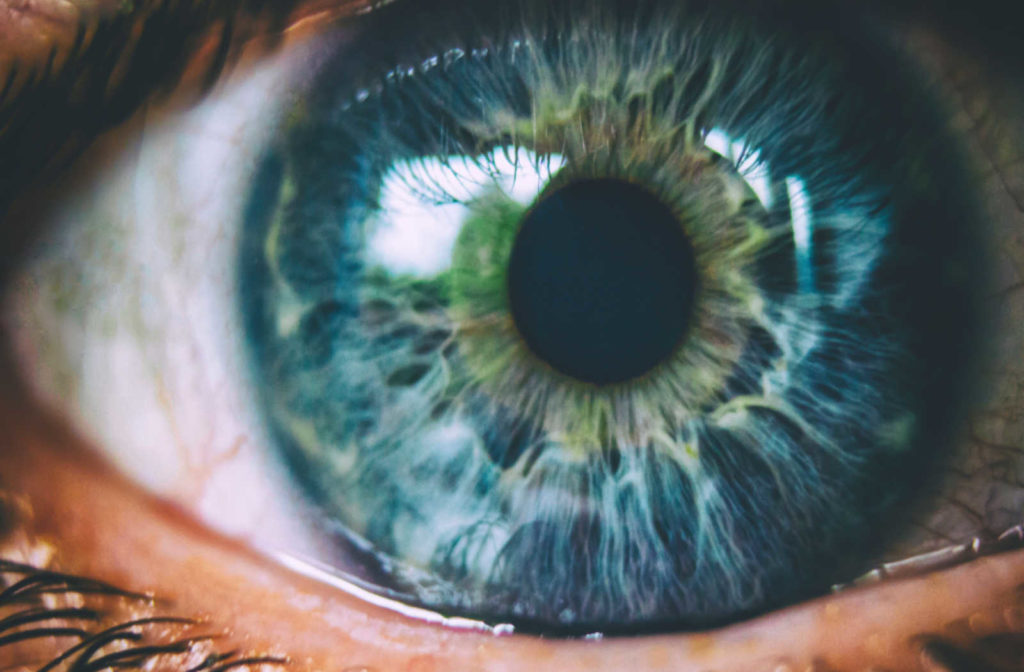This photograph is an extreme close-up of an eye, prominently featuring the intricate details of the iris and pupil. The iris is primarily a deep blue, reflecting shades of green from possibly a nearby tree, adding layers of color to the image. The pupil is centered slightly to the right, creating a focal point that draws the viewer's gaze. The eye is surrounded by subtle shades of white and peach representing light-colored veins, with black and brown hair sprouts around the eyelid area. The rectangular image captures every nuance, with eyelashes visible at both the top and bottom of the frame. The overall setting is the detailed anatomy of the eyeball, and there is no text present in this vivid and realistic photograph.